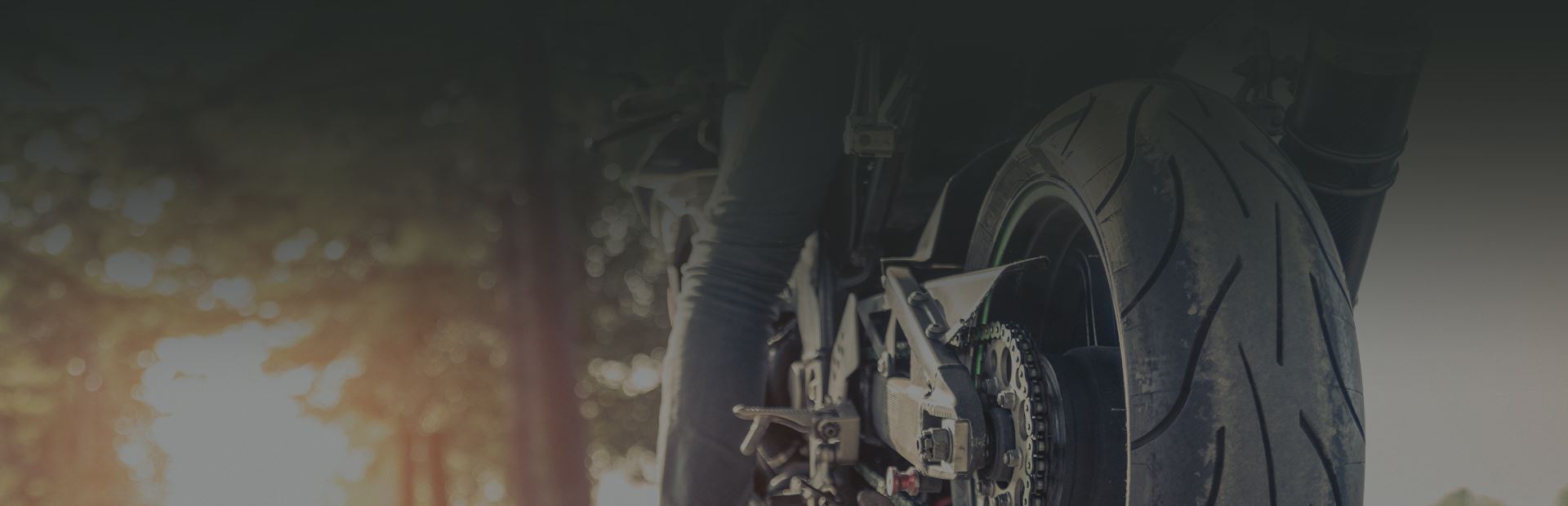The photograph is a professionally shot, artistic close-up of the rear tire of a motorcycle, taken from a low angle almost at ground level. The focal point is the back tire and its intricate details, including the gears and the chain. The image captures the straight leg of a person, clad in blue jeans, hanging to the side of the motorcycle, while the other leg is hidden due to the angle. Part of the motorcycle's exhaust pipe is visible on the right side, although it is partially cropped. The background is softly blurred, providing a depth of field that contrasts with the sharply focused foreground. In the backdrop, a tall tree with green and yellow leaves is visible against an orangish, muted sky, indicating a sunset. The photograph has been edited with desaturated colors, adding to its artistic feel. The image is significantly wider than it is tall, emphasizing the elongated perspective of the motorcycle and its surroundings.